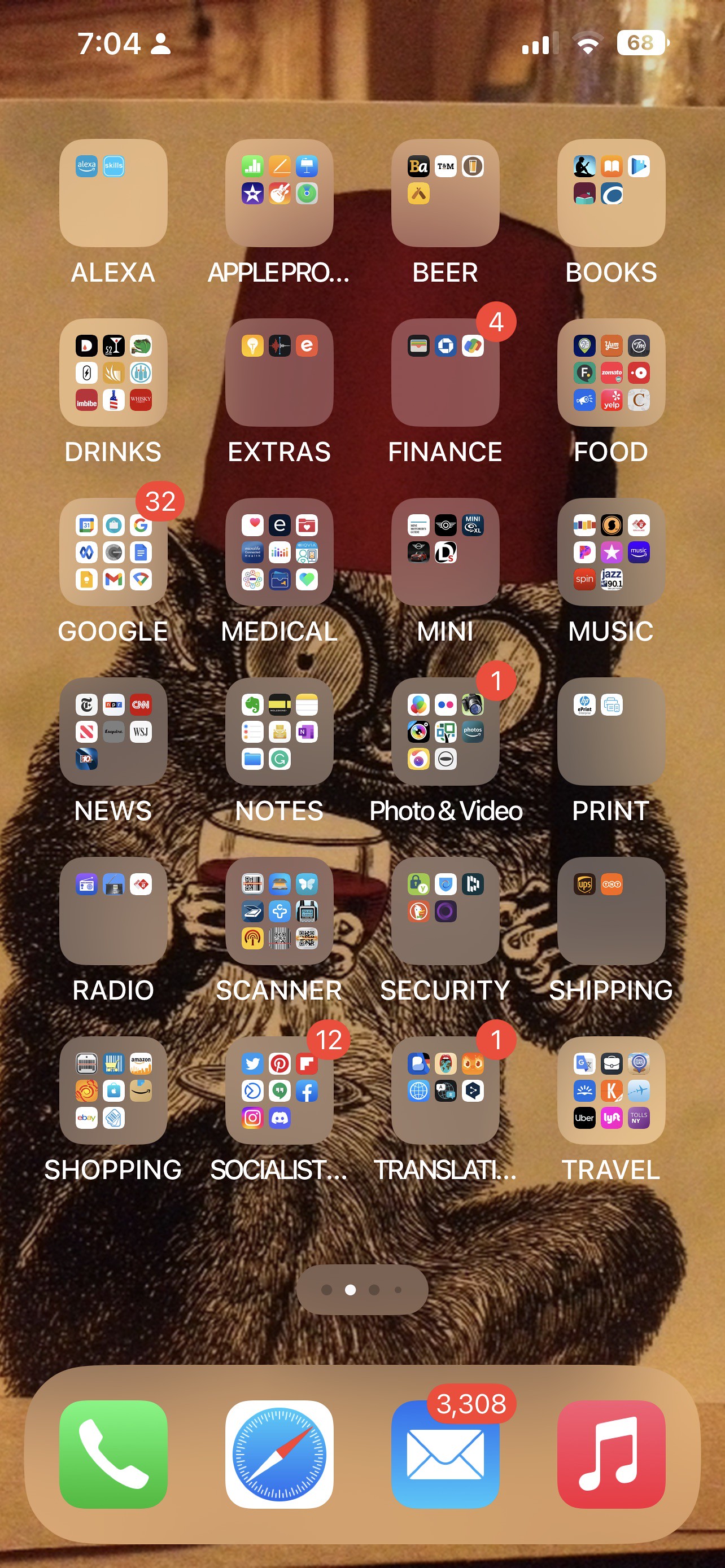This image is a detailed screenshot of a mobile phone's user interface, showcasing various menu items and status indicators. At the very top of the screenshot, the status bar displays several elements. On the left, in white text, is the time "7:04" with a person icon next to it. On the right, there are three white bars indicating mobile signal strength, followed by an icon depicting Wi-Fi signal strength with two curved lines, and lastly, the battery percentage, "68%", also in white.

The bottom of the screenshot features four main menu icons. The first icon on the far left is a green background with a white telephone symbol, representing the phone app. Next to it is the compass app, illustrated by a blue circle with red and white directional hands. The third icon is for the email app, depicted by a white envelope on a blue background with rounded edges, notably showing "3,308" unread messages in red text. The last icon on the right is for the music app, featuring two white quavers (musical notes) on a red background.

The wallpaper of the phone displays an intriguing sketch of a furry creature with claws and large eyes. The creature dons what appears to be a red hat resembling Freemason's headgear or an upside-down bowl.

Six rows of app folders appear in the main menu section, each organized by category. The top-left folder is labeled "Alexa" containing various Alexa apps or widgets. To its right, the next folder "Apple Pro" shows smaller icons indicating six items within. The following folder has a label "Beer," suggesting it contains apps related to that category. Each folder icon showcases a minimalist design highlighting its purpose clearly.